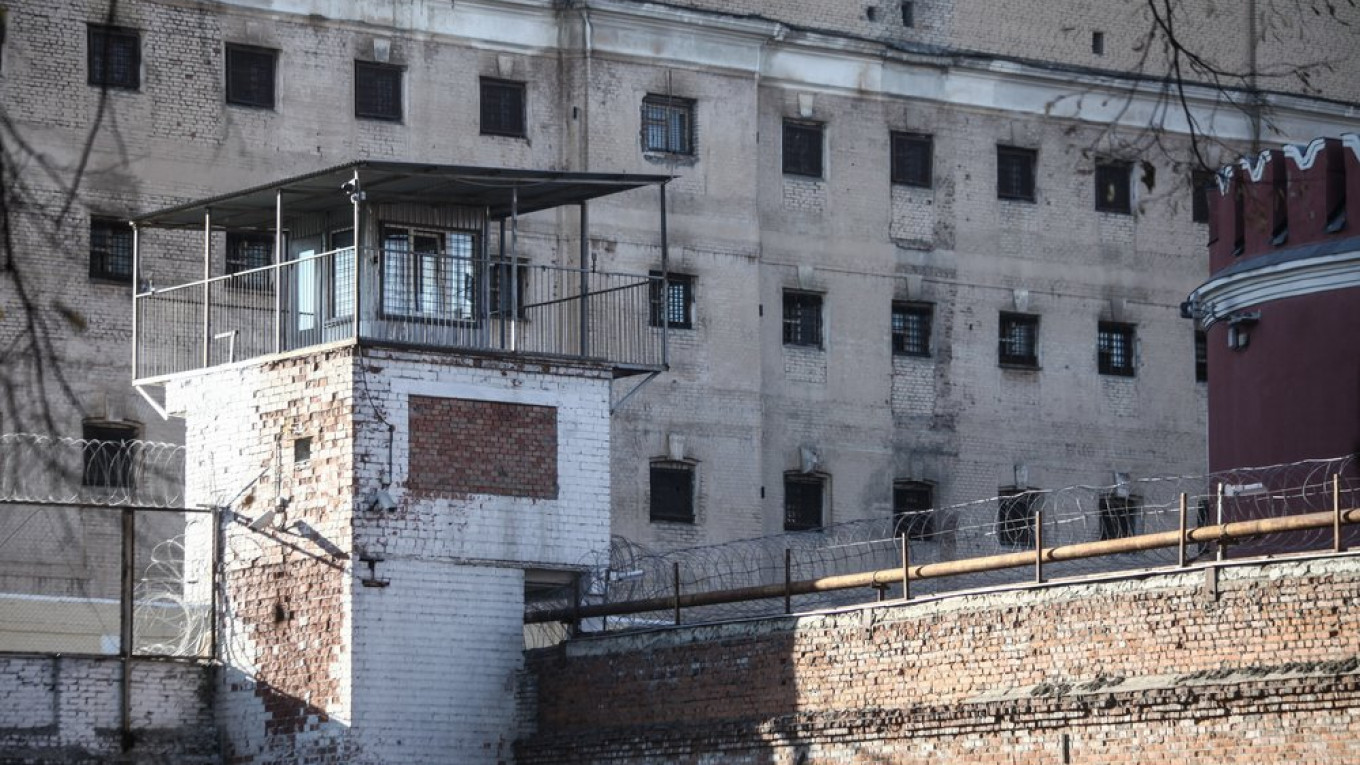The photograph captures an angled view of a dilapidated and likely abandoned prison complex during the daytime. Dominating the left side of the image is a white brick guard tower with peeling paint, topped by a guard shack surrounded by a gray fence. Adjacent to this, a barbed wire-topped metal fence extends into the image's left corner. Moving right, a long stone wall, also topped with barbed wire, runs parallel to a grim-looking stone complex that features multiple rows of small, square windows, each covered with black bars. Further into the background, another prominent structure made of red brick with white accents at the top stands out, adding to the somber atmosphere. The complex appears weathered and forlorn, emphasizing its deserted and eerie aura.